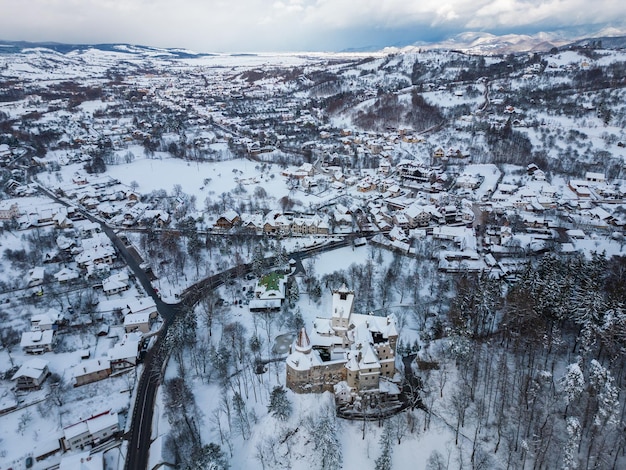This aerial photograph, likely taken by a drone or helicopter, captures a picturesque winter scene in a small European town nestled in the snow-covered hills. At the center bottom of the image, a large, stone castle or church stands prominently, its towering structure contrasting against the surrounding landscape. A curved road enters the frame from the bottom left, splitting into a triangular formation before winding towards the middle of the image, and then diverging towards the left. This network of roads is bordered by numerous small houses, their rooftops blanketed in snow, creating a patchwork of white over the brown and gray structures.

Interspersed among the houses are clusters of trees, their dark tones adding depth to the snowy terrain. The overall color palette of the scene is a mix of stark whites, off-whites, browns, dark grays, and occasional hints of green, giving the landscape a rich, textured appearance. The top of the image reveals a strip of blue sky veiled by an expanse of white clouds, emphasizing the daytime setting. The snowy landscape, detailed buildings, winding roads, and scattered trees together create a serene yet intricate winter tableau, reminiscent of a historic European village.